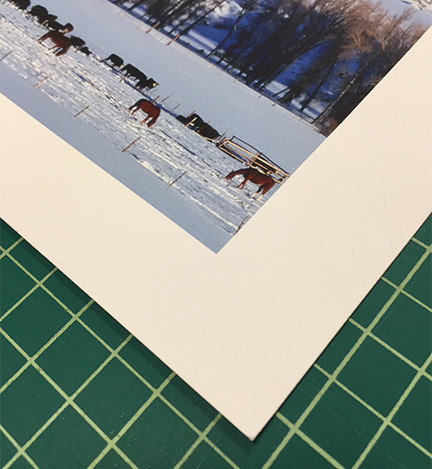The image shows the bottom right corner of a photograph resting on a green checkered surface with light green lines forming a graph-like pattern against darker green tiles. The photograph itself features a wintery farm scene: several chestnut brown horses and possibly black cows are standing and lying in a snow-covered field that has been disturbed by their movements. The animals are grazing near a barn, and there are visible fence posts in the foreground. In the background, barren trees and distant mountains emerge from the snowy landscape, adding depth to the scene. The photograph is bordered by a thick white frame, around two to three inches wide.